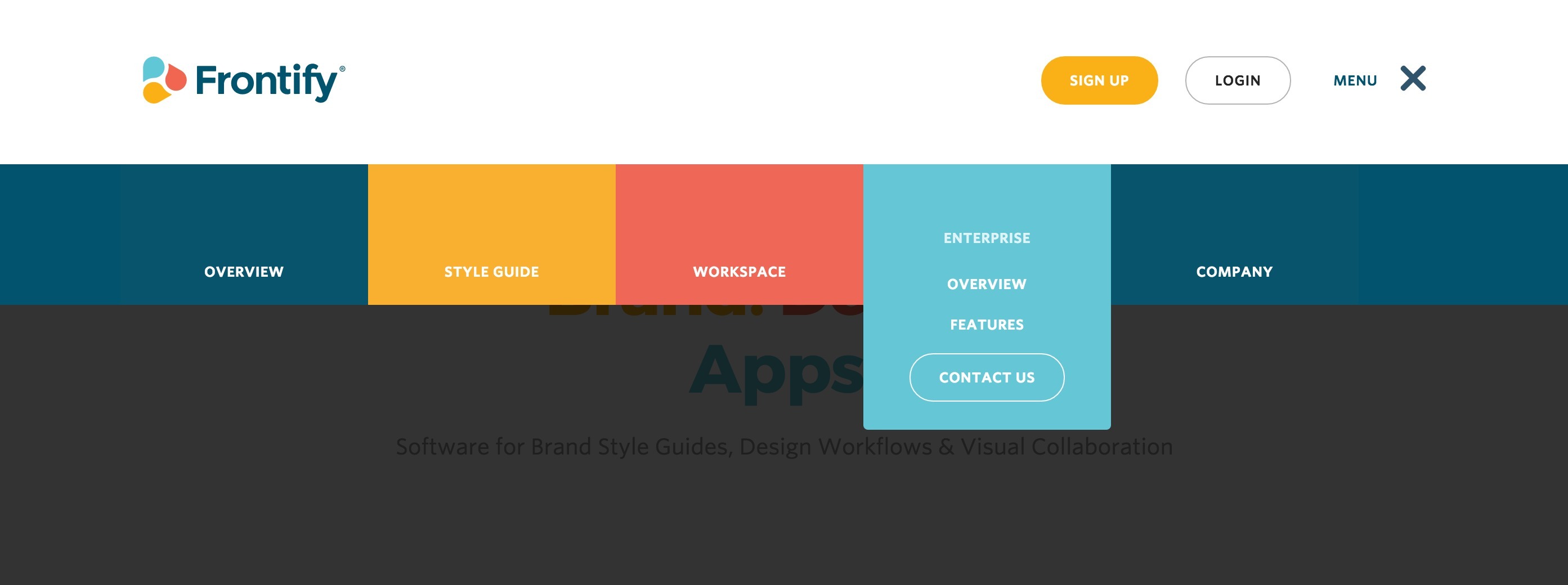This image captures the top section of the Frontify website, showcasing its logo and navigation elements. The Frontify logo, located at the top left corner, is a geometric design featuring a triangle composed of turquoise, yellow, and pinkish-red teardrops. Adjacent to the logo on the top right corner are three buttons: a yellow "Sign Up" button, a white "Log In" button, and a "Menu" button in dark blue text, followed by a small blue 'X'. Below these buttons, a multicolored menu bar spans horizontally across the top section, with each segment representing different site sections: a dark blue segment for "Overview," a mustard yellow for "Style Guide," a reddish pink for "Workspace," light blue for "Enterprise," featuring dropdown options like "Overview," "Features," and "Contact Us," and finally, another dark blue segment for "Company." The use of vibrant colors and clear labeling establishes an organized, visually appealing interface.